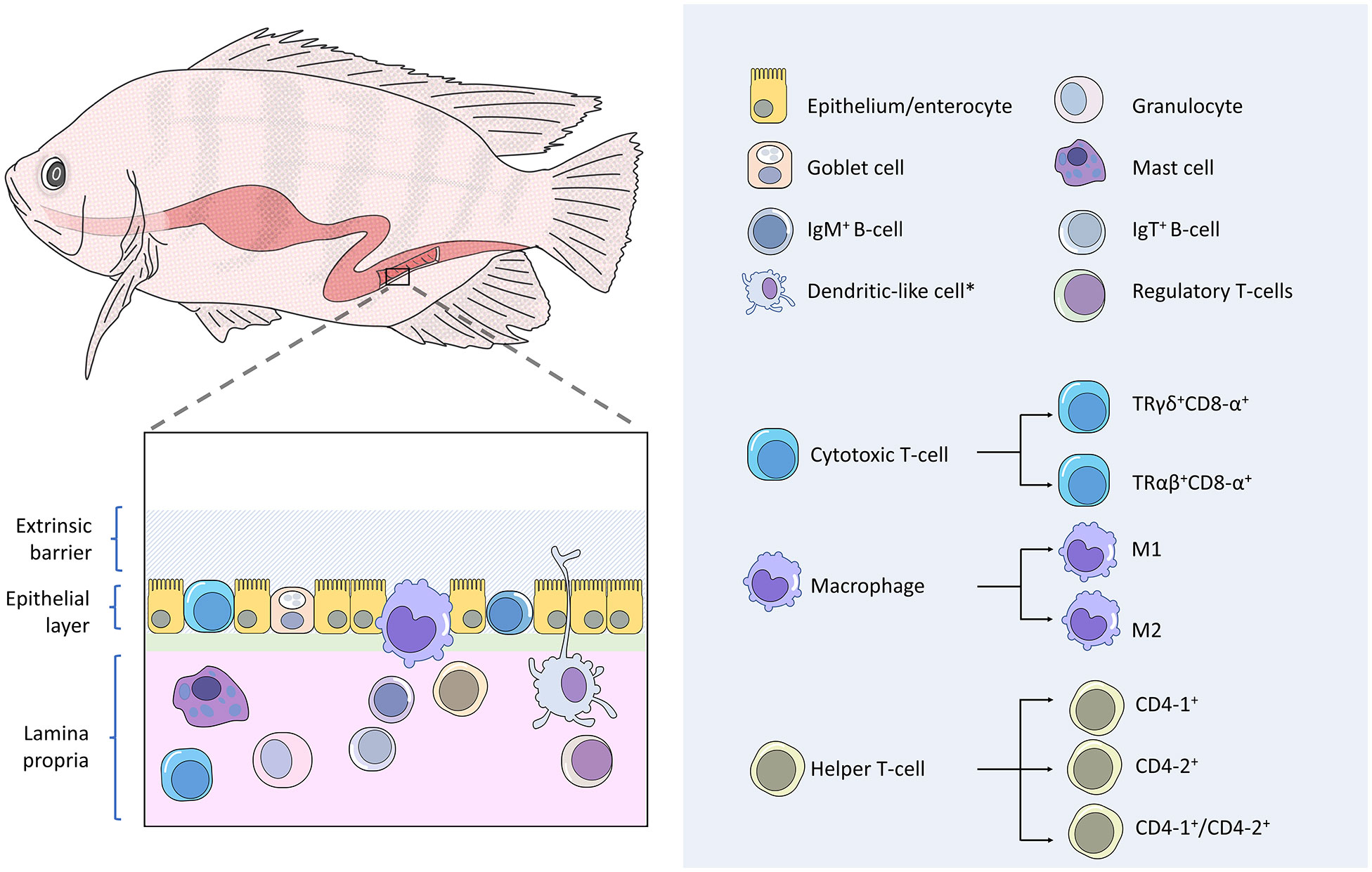This intricate scientific diagram details the anatomical and cellular composition of a fish, focusing particularly on the fish's skin. In the upper left-hand corner, a mauve-colored fish with a red stripe is depicted, illustrating the point of study. Directly beneath this fish is a magnified view of its epithelial layer, the outermost skin, detailing the underlying lamina propria. The diagram uses a palette of yellow, gray, white, and purple to denote various structures. To the right, there is a comprehensive table and explanation chart that catalog the different cells present in the fish’s skin, including epithelial cells, enterocytes, granulocytes, mast cells, goblet cells, IgM+ B cells, dendritic-like cells, regulatory T cells, cytotoxic T cells, macrophages, and helper T cells. This section serves as a legend to better understand the diagram, providing detailed descriptions of each cell type and their roles. This informative flowchart effectively breaks down the fish's skin to a microscopic level, elucidating the complex interplay of cells and barriers within.